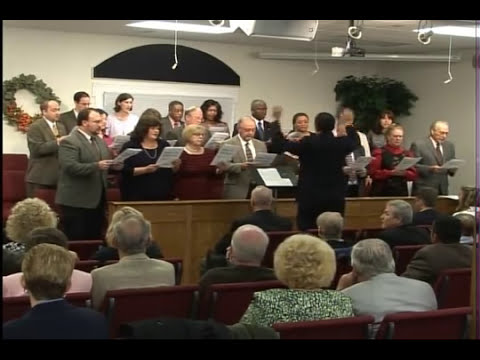The image depicts a choir performance taking place in a church adorned with festive Christmas decorations. There are around 20 members in the choir, comprising older men dressed in suits and ties and women in formal dresses, all holding sheet music. The conductor, clad in a black suit, stands with his arms raised, facing the choir with his back to the audience, which consists of older, elegantly dressed individuals seated in red chairs.

The background walls are white, and to the left, a Christmas wreath with red bows is prominently displayed, suggesting the season. Directly opposite, on the right, is a large Christmas tree. There is a black-awninged window visible in the background, with lights and white cords descending from the ceiling. Additionally, there is a black plaque on the wall, though the text is unreadable. The overall ambience suggests an indoor setting with a festive, seasonal theme, likely hinting that the choir may be performing Christmas carols.